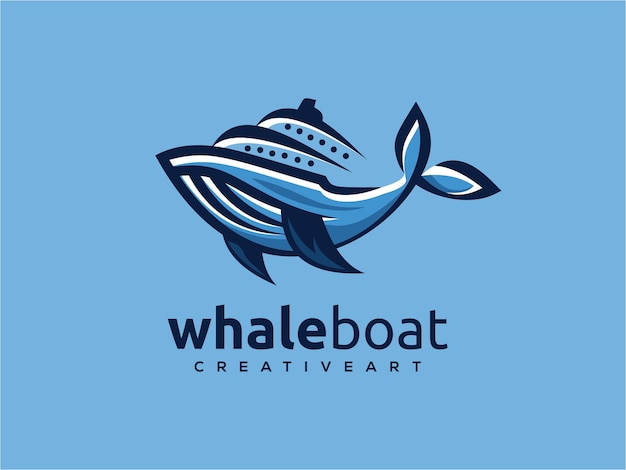The logo image features a unique and creative design on a light blue rectangular background. Central to the logo is the word "whaleboat" in a distinctive font: "whale" is bolded and in navy blue, while "boat" is non-bolded but connected, both sharing the navy blue color. Below "whaleboat," in a smaller plain black font, are the words "CREATIVE ART" in all caps. 

Above the text is a stylized and simplified depiction of a whale, composed of shades of navy blue, light blue, and medium blue. The whale's fins are notably darker, with the entire body showcasing the underside and tail. Integrated into the whale's back is the upper structure of a steamboat or luxury cruise ship, complete with several portholes and what appears to be a smokestack, blending together the elements of a whale and a boat seamlessly to visually represent the "whaleboat" concept. The cohesive design signifies a company likely named "Whale Boat Creative Art," combining marine and nautical themes in a visually appealing manner.